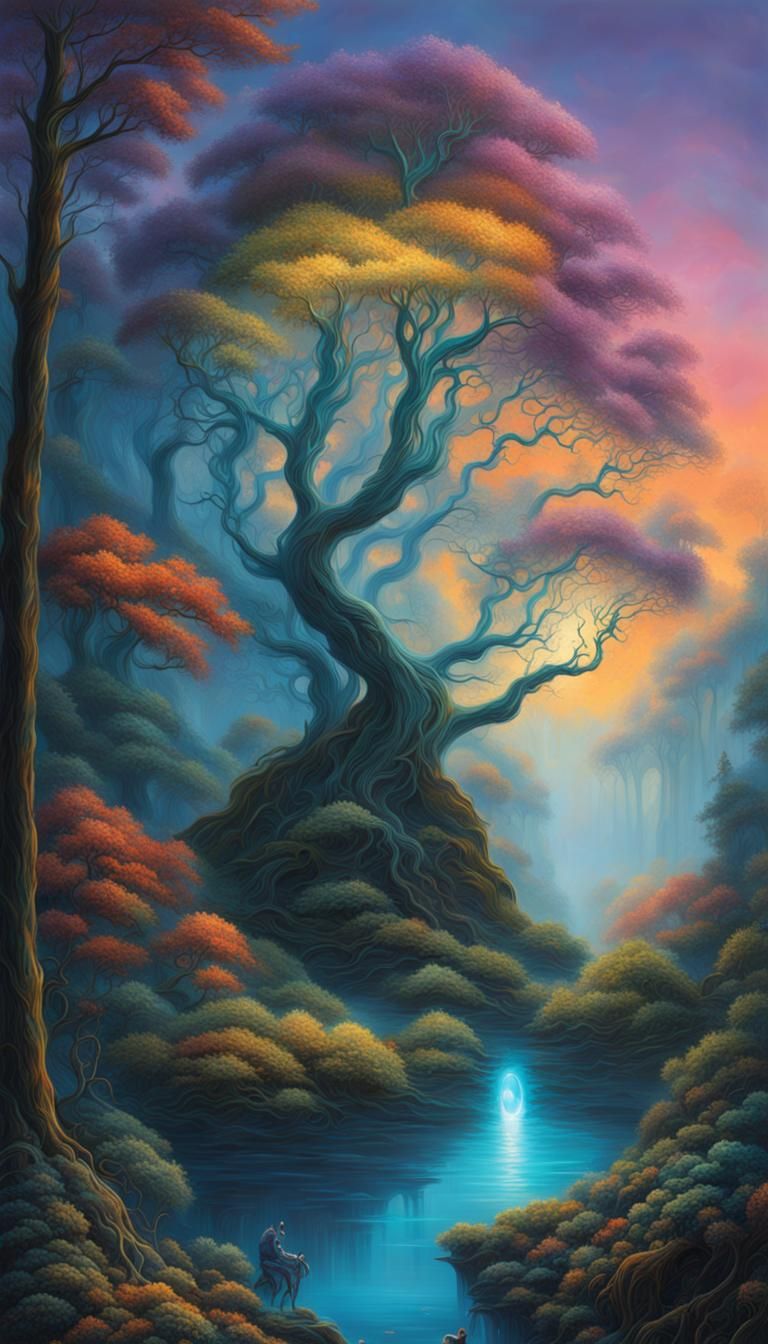This image showcases a beautiful, artistic painting centered around a massive, enchanting tree. The tree dominates the scene with its wide, prominently winding roots that transition into an intricate trunk, and numerous, large, squiggled branches. Its foliar canopy boasts a spectrum of purplish-pink, orange, yellow, and reddish leaves that are round and bushy, creating a vibrant display particularly towards the top and right side of the tree.

The foreground of the image features a serene, bright blue waterway, with a glowing blue orb illuminating the scene near the tree. Towards the bottom left, a small horse stands near brightly colored bushes, adding a sense of scale and life to the composition. Smaller trees with orange tufts and various foliage line the banks of the waterway, echoing the design of the giant tree but on a lesser scale.

In the background, more trees create a layered depth, showing leaves that are primarily red and blending into the vivid and dynamic sky. This sky transitions from a warm yellow and orange hue at the horizon into shades of pink, purple, and ultimately a light blue at the zenith, enhancing the painting’s dreamlike quality. The combination of these elements forms a striking and detailed portrayal of a fantastical natural landscape.